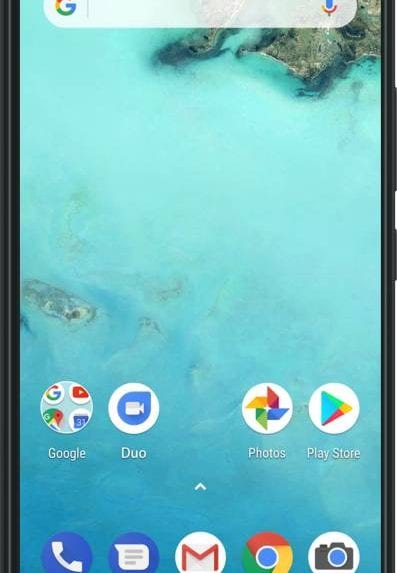The image showcases a mobile phone home screen with a variety of apps and features prominently displayed. At the top, there is a Google search widget containing a microphone icon for voice search on the right side. Below the search bar, a folder is visible which houses several Google apps including Google, YouTube, Google Maps, and Google Calendar. Other apps on the home screen include Google Duo, Google Photos, Google Play Store, Phone, Messages, Gmail, Google Chrome, and Camera. The wallpaper is a vibrant mix of blue, green, red, yellow, white, and grey, adding a colorful background to the neatly arranged icons.